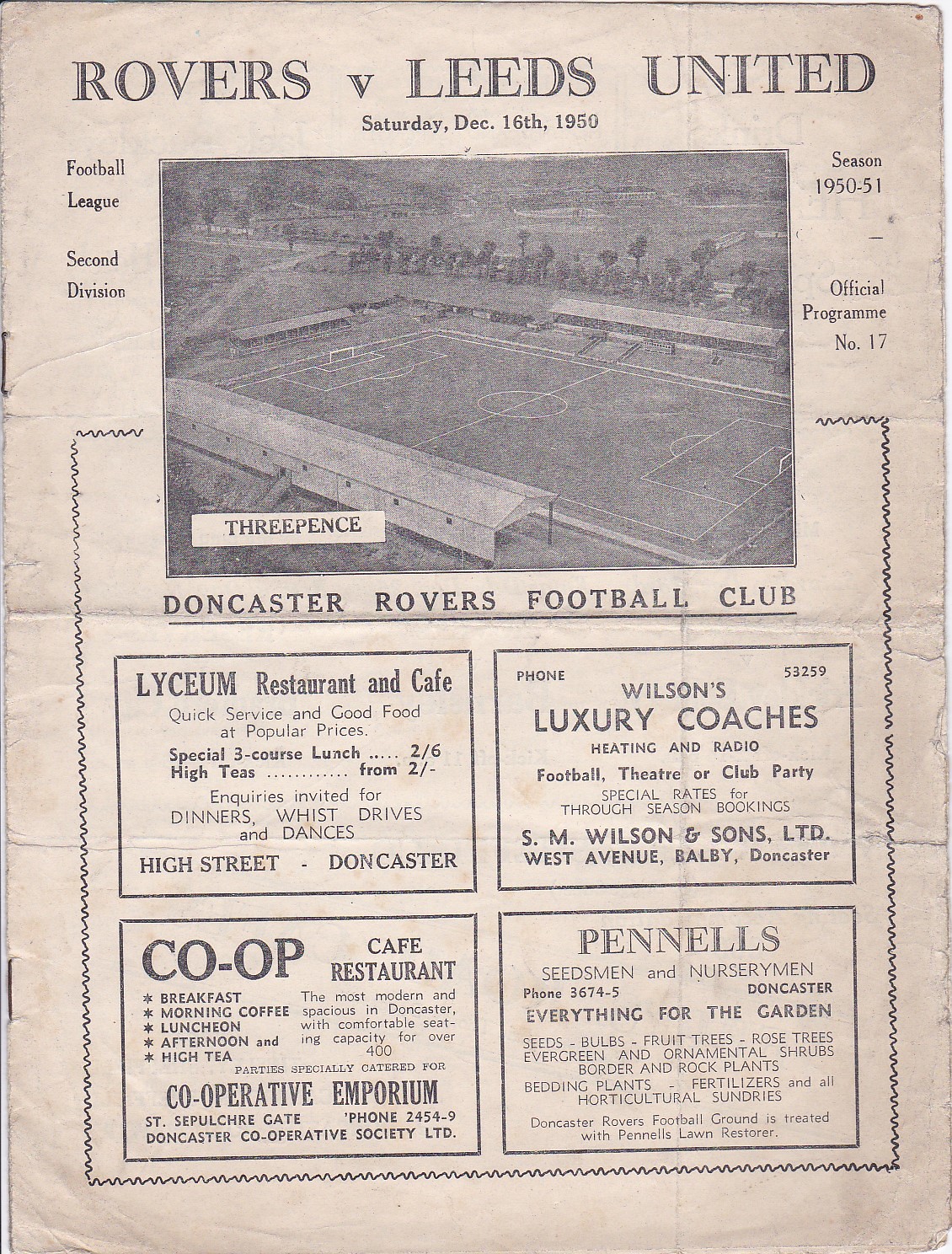This vintage, crumpled, and folded sports program from December 16th, 1950, encapsulates the history and atmosphere of mid-20th-century football. Yellowed with age and marred by cracks and rusty staples along its left binding, it evokes a deep sense of nostalgia. Titled "Rovers versus Leeds United," for a Football League Second Division match during the 1950-51 season, it proudly announces itself as the official program number 17, priced at three pence.

Dominating the page is a faint black-and-white aerial photograph of a soccer field, beneath which the bold text "Doncaster Rovers Football Club" stands out. Complementing the historical ambiance, the bottom section contains four distinct advertisements framed in thin black lines. 

To the left, the Lyceum Restaurant and Cafe promises quick service and quality food at popular prices, boasting a three-course lunch, high teas, dinners, and facilities for drives and dances, located on High Street, Doncaster. Next, Wilson's Luxury Coaches, with the contact number 53259, offers heated and radio-equipped transport for football, theater, or club parties, managed by SM Wilson and Sons Limited, West Avenue, Balby, Doncaster.

On the right, Pinnell's advertises its services as seedsmen and nurserymen with contact numbers 3674-5, providing everything for the garden including seeds, bulbs, fruit trees, rose trees, bedding plants, and horticultural sundries. They proudly state that Doncaster Rovers' football ground is treated with Pinnell's Lawn Restorer. Finally, the Co-op Cafe Restaurant, run by the Doncaster Cooperative Society Limited with the phone number 2454-9, describes its modern and spacious venue in the Cooperative Emporium, accommodating over 400 guests and offering breakfast, morning coffee, lunch, and afternoon high tea, with a particular emphasis on parties.